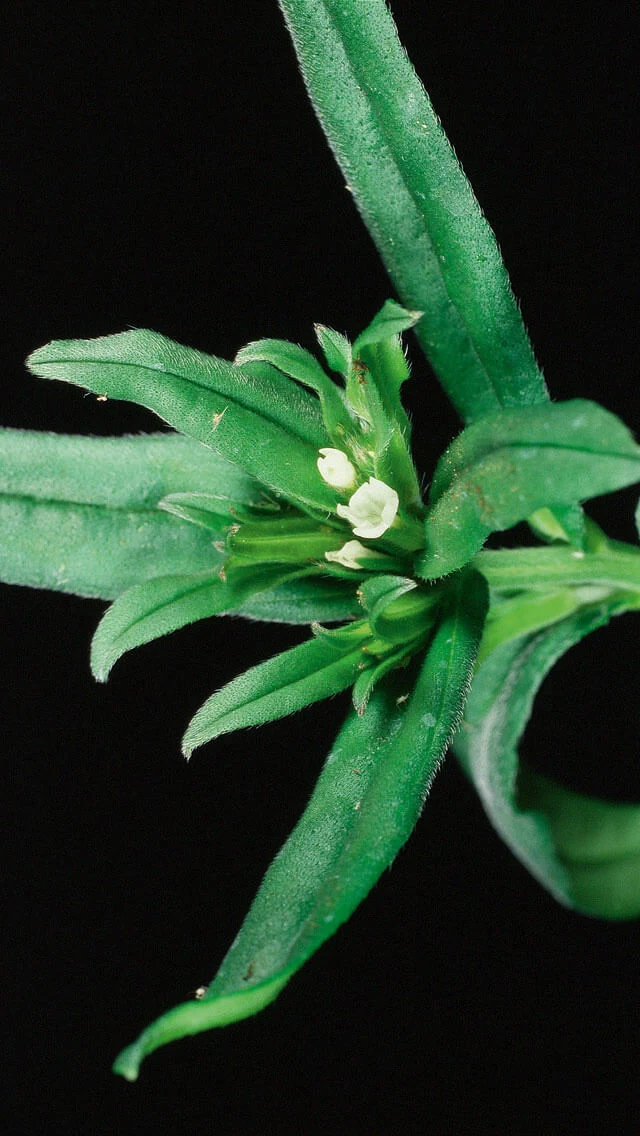This vertical rectangular image is set against a black background, capturing a close-up of a green plant. The plant features a complex arrangement of stems and leaves, with some stems extending horizontally across the middle of the image and others going in various directions. One large stem extends upward, while another prominent leaf reaches down toward the bottom left corner. Surrounding these are multiple green leaves, including about six or seven prominent ones and several smaller, narrower leaves clustered in the center. The image's focal point lies in the middle, where three tiny, circular white blossoms are visible. One blossom is open, revealing a hint of green at its center, while the other two remain closed. The shorter leaves nearby appear curled, straightening out as they grow longer. The intricate details of the plant's structure and the delicate white flowers stand out vividly against the dark backdrop.